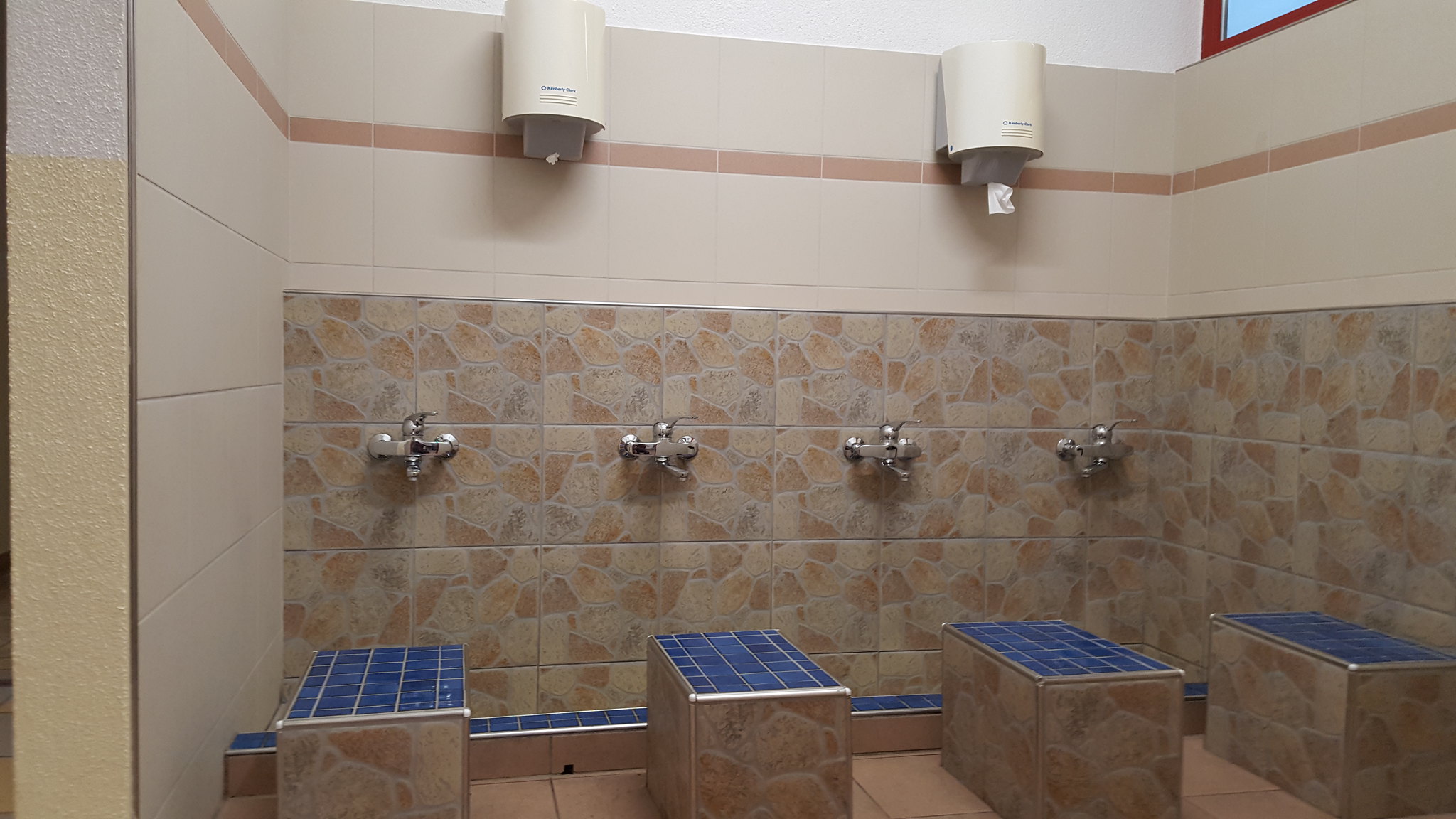The image depicts a sit-down shower area, possibly of Japanese origin, often featuring communal shower setups. The setting encloses a tiled environment, with a distinctive variegated pattern of brown and gray stone tiles forming four benches. Each bench is topped with beautiful small blue tiles, echoing a similar blue trim that outlines the trough running along the foot of the structure. Above these benches, four silver metal faucets are mounted slightly lower on the wall, likely intended for people to sit and wash rather than standing as in a typical shower setup.

The back wall features a light off-white, beige tile with a brown border, offering a contrast to the variegated tiles below. Above the faucets and benches, a beige stone tile is capped by a thinner strip of tan tile, leading up to a higher portion of the off-white wall. In this upper section between the first two and the last two faucets, there are white dispensers that possibly provide towels or soap. Additionally, there's a hint of a window's edge in the far upper right corner, lending a touch of natural light or openness to the otherwise enclosed space.

Overall, the combination of practical fixtures and aesthetically pleasing tile work suggests a well-thought-out design meant for both functionality and a soothing wash experience.